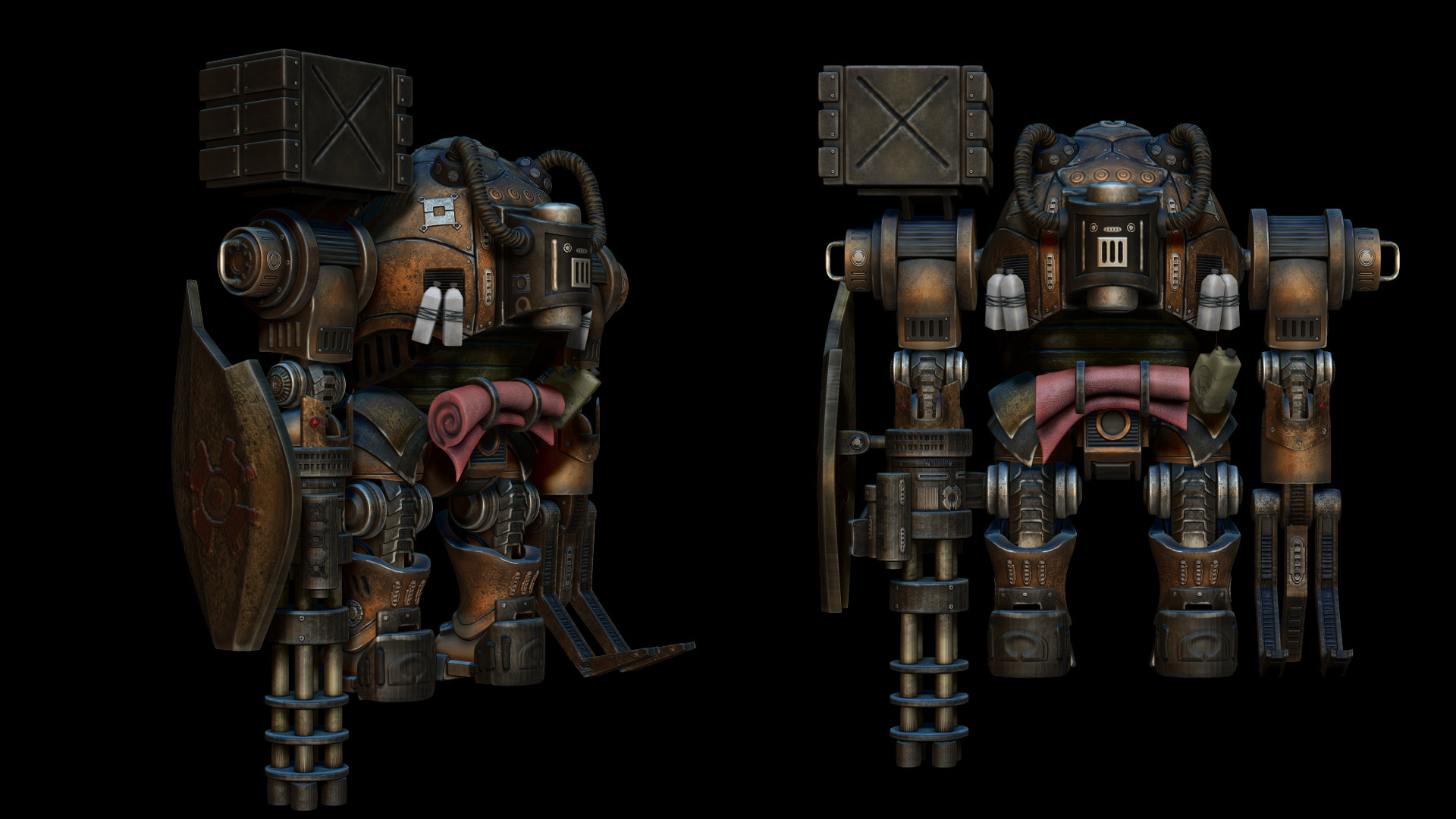In this detailed rendering, there are two steampunk-inspired robots standing against a completely black background. Both robots are predominantly metallic, adorned with brown and brass hues that gleam under the focused lighting. They appear chunky and robust, each having a distinctive design that evokes imagery of machines depicted in computer games or vintage submersibles.

The robot at the forefront is facing directly towards the viewer, showcasing a formidable appearance with features resembling a slot machine but devoid of any typical slot machine graphics. Its right arm is replaced by an imposing Gatling gun with six barrels, exuding a menacing presence. Mounted on top of the Gatling gun is a large box marked with an X, reinforcing its mechanical and steampunk aesthetic. The robot also has several white bottles and metal barrels with hooks protruding from its sides, adding to its complex design. A rolled-up object, appearing like a towel or pad, is noticeably situated on its front, suggesting some functional purpose.

The second robot, positioned slightly to the side, shares a similar build but offers a different perspective - a mix between a straight-on and isometric view. This vantage point reveals not just the Gatling gun on its arm but also a protective shield surrounding it. Both robots feature streamlined, cylindrical legs mounted on simple hinges, allowing movement in a single direction, further emphasizing their mechanical nature.

These intriguing creations merge the aesthetics of steampunk with functional design elements, making them appear as if they have stepped out of a fantastical, mechanized world.